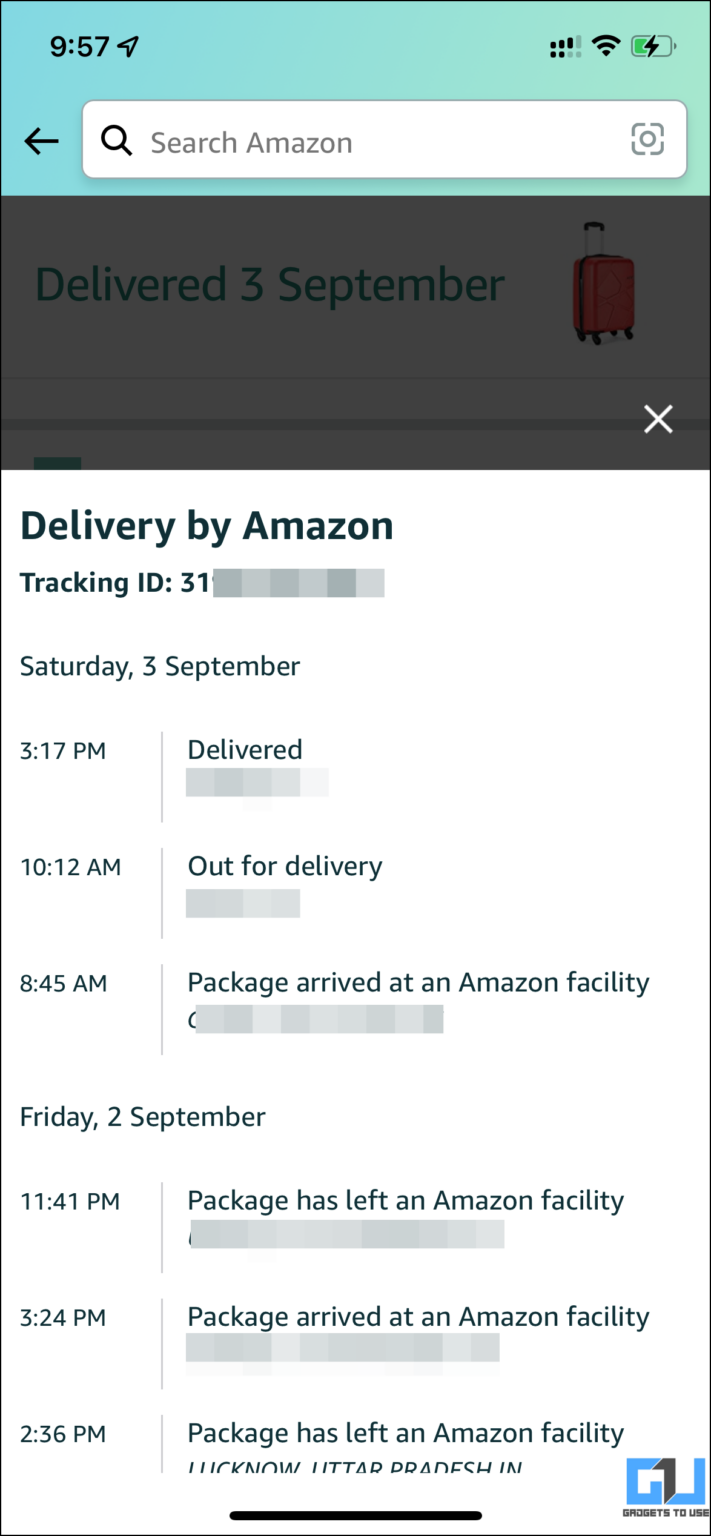The image depicts a screenshot of an Amazon delivery tracking page on a smartphone. The phone, currently charging, displays the time as 9:57 in the top-left corner. A teal-colored strip is situated at the top of the screen. Below this strip, a white search bar prominently displays the text "search Amazon."

The main content area features a dark overlay box that provides details of a recent delivery. In the background, faint but discernible text reads "delivered 3 September." The item delivered appears to be a red rolling suitcase with extended handles and four wheels. A small white X is located at the top-right corner of this dark overlay box.

The next section of the screenshot, beneath the dark overlay, shows bolded text stating "delivery by Amazon." Below this, it mentions a partially obscured tracking ID: "3 1 —— —— —— —— ——," where some numbers are either blacked out or grayed out. The text "Saturday, 3 September" is listed below the tracking ID, followed by a detailed log of the package's journey:

- **3:17 PM**: Delivered (information below is grayed out)
- **10:12 AM**: Out for delivery (information below is grayed out)
- **8:45 AM**: Package arrived at an Amazon facility (information below is grayed out)
  
For the previous day, **Friday, 2 September**:
- **11:41 PM**: Package has left an Amazon facility (information below is grayed out)
- **3:24 PM**: Package arrived at an Amazon facility (information below is grayed out)
- **2:36 PM**: Package has left an Amazon facility, with the noted location "Lucknow, Uttar Pradesh, IN."

At the bottom right of the image is an icon with the text "Grogets to use," featuring a blue "G" and a gray and white "U" logo above it.